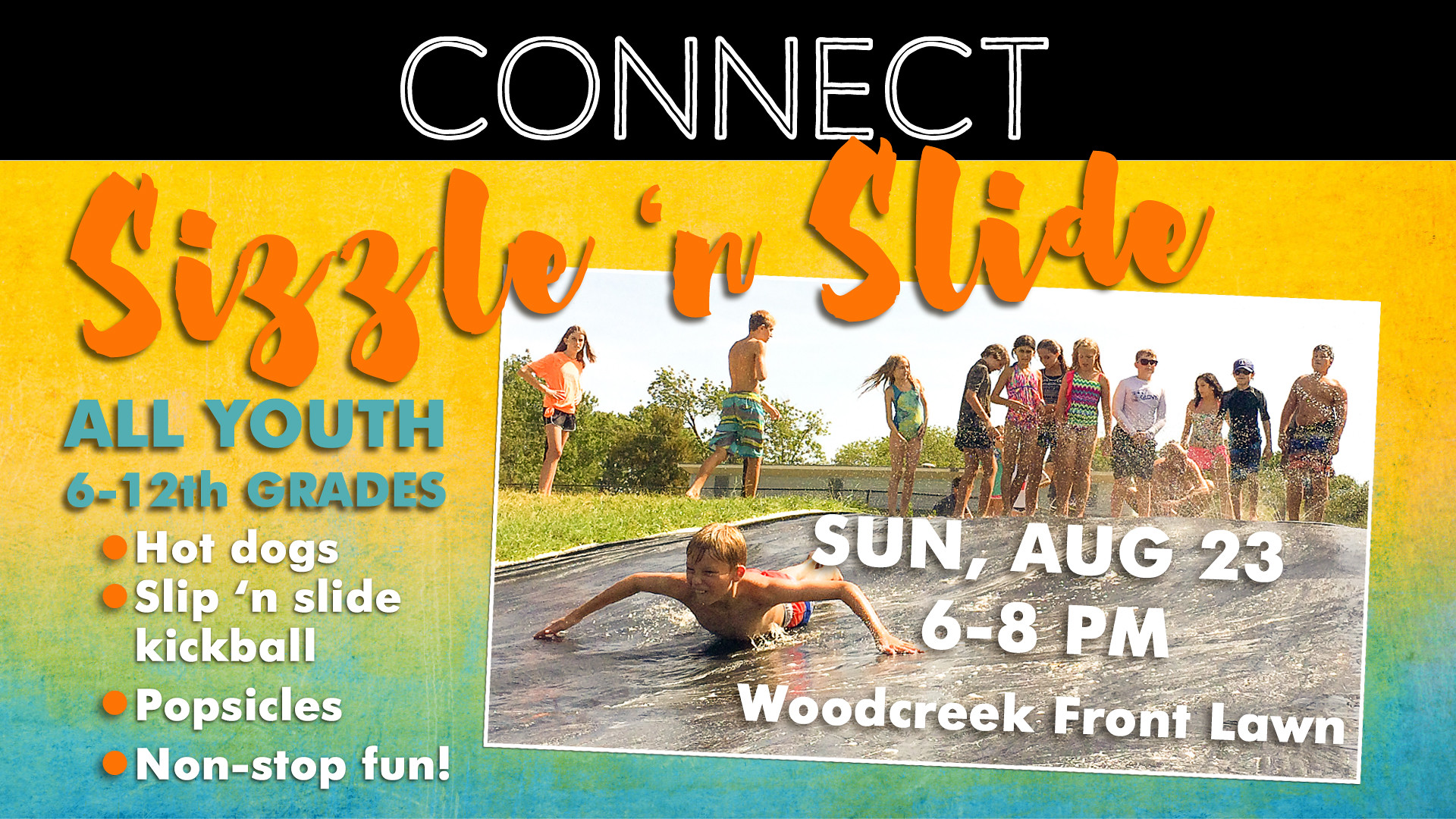The landscape-oriented flyer for a youth event features a vivid blend of photographic and graphic elements. Dominating the top fifth of the flyer is a black header with the word "CONNECT" in white text, intricately outlined to create a dual tone effect. Beneath the header, the background transitions in a gradient from golden yellow at the top, to green, and finally to blue at the bottom. Diagonally across the yellow portion, in an eye-catching orange script, is the event title "SIZZLE AND SLIDE."

On the left side, blue text announces "ALL YOUTH 6th to 12th grades." Directly below this, four orange bullet points highlight key activities: "HOT DOGS, SLIP AND SLIDE, KICKBALL, POPSICLES," and particularly emphasizing "NON-STOP FUN." On the right side, there’s a vibrant outdoor photograph showing children enjoying a slip-and-slide on a grassy lawn, with some kids actively sliding and others waiting in swimwear. Overlaid on this image, white text provides essential event details: "Sunday, August 23rd, 6 to 8 p.m., WOOD CREEK FRONT LAWN." The diverse color scheme includes black, white, orange, blue, green, and yellow, merging realism with stylistic typography to create an engaging and dynamic promotional flyer.